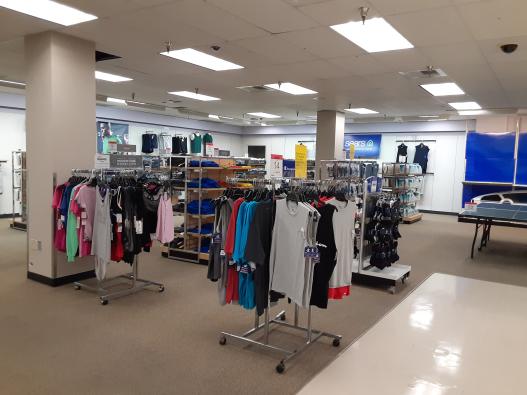The image depicts the interior of a clothing store with several notable features. The store is illuminated by rectangular fluorescent lights embedded in the ceiling, and there are visible sprinklers and cameras. The majority of the floor is covered with light brown carpeting, but the bottom right corner reveals a section of shiny white tiles. Two prominent support beams stretch from floor to ceiling. On the left side of the image, multiple racks are organized with various styles of clothing, including pink, blue, and white dresses, alongside tennis and longer dresses. Price tags are visible on the racks. The right side of the image features a blue tarp covering part of the wall, possibly acting as a cover for a pinball or ping pong table situated in front of it. Mannequins dressed in black garments and additional merchandise can be seen behind the clothing racks. The store has a predominantly neutral color scheme with white walls and a gray section of the floor, creating a clean and organized retail environment.